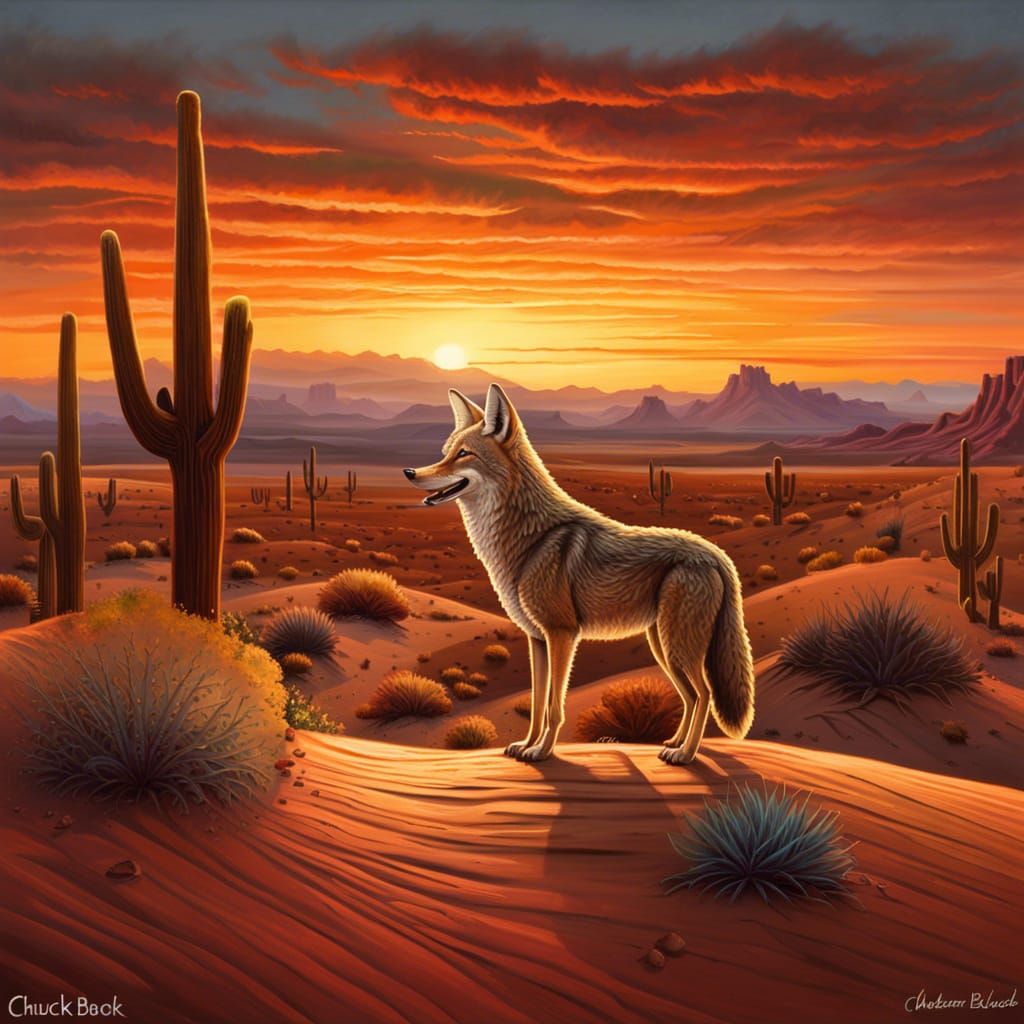The painting depicts a captivating desert scene during what appears to be either sunrise or sunset, as suggested by the sky's gradient of varying orange hues. At the bottom left-hand corner of the artwork, the words "Check Back" are inscribed in white. Contrasting this, the bottom right-hand corner bears a distinct signature, also in white, with the initials "CB," though it seems to belong to a different name. The scene is dominated by a grayish-white coyote positioned on arid, reddish-brown terrain, gazing towards the left. Surrounding the coyote are scattered cacti, adding to the rugged atmosphere. The desert landscape features a mix of brown, reddish, and orange tones, and is framed by distant mountains, enhancing the desolate yet beautiful setting. The sun, positioned low on the horizon, contributes to the dramatic and atmospheric lighting of the painting.